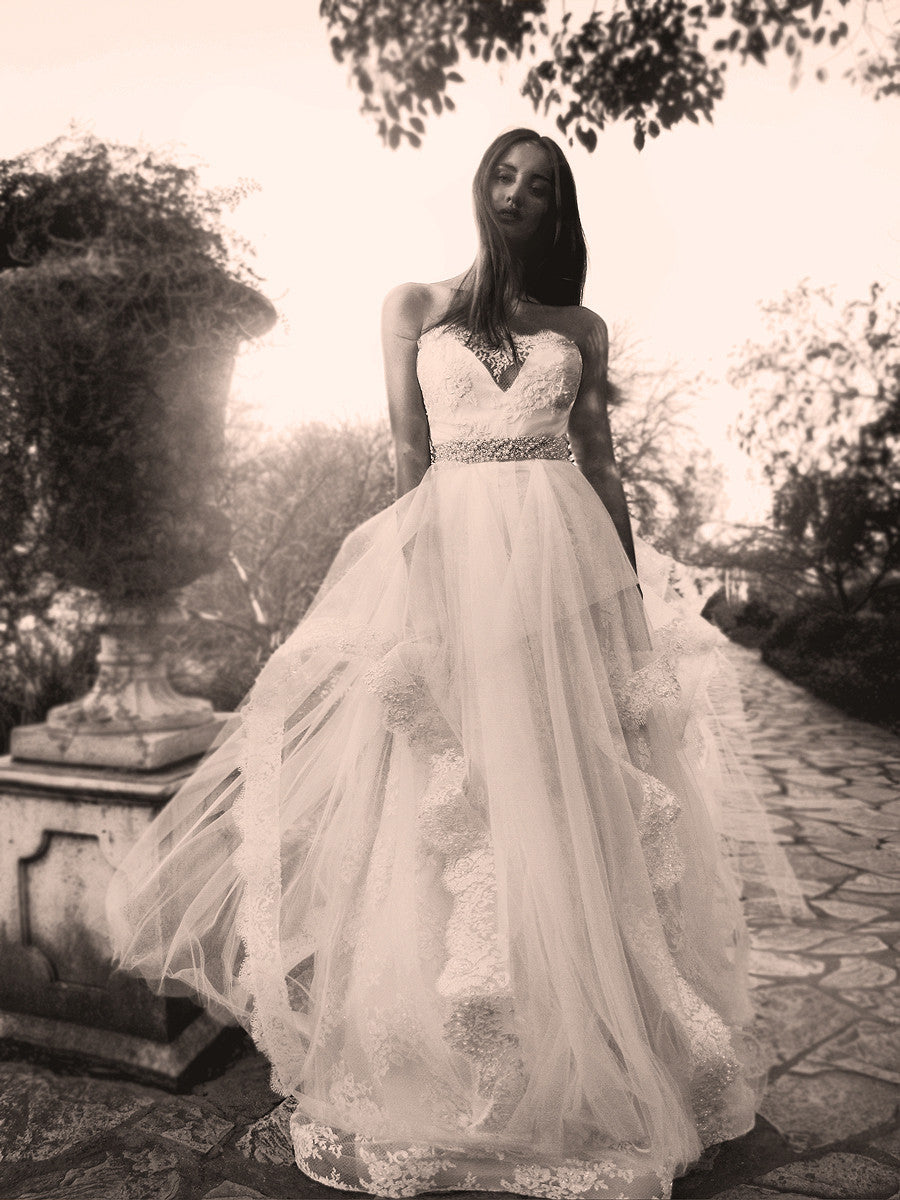In this black and white photograph, a young woman in her early to mid-20s poses in a stunning wedding dress on a cobblestone pathway, framed by the lush greenery of a garden. Her light brunette hair cascades to just below her shoulders, with the right side tucked to the front and the left side flowing behind her back. The dress is a strapless, form-fitting gown with a deep V cut in the center, adorned with a silver belt at the waist and a flowing sheer tulle skirt embroidered with delicate floral designs. Her expression is neutral and serene, as she gazes directly into the camera. To her right, a decorative stone chalice overflows with entwined vines and leaves, adding a whimsical touch to the scene. Above, tree branches extend, their leaves visible in the frame, while the distant sun adds a soft backdrop to this timeless moment. Despite being in what seems to be a lively wedding venue, she stands alone, creating an intimate, peaceful atmosphere.